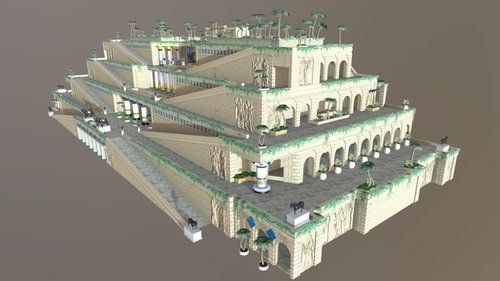This is a computer-generated 3D model depicting a large, four-story compound building with a Middle Eastern architectural style. The building is predominantly white with gray floors and is set against a gray background. The structure features numerous arches on the second, third, and fourth levels, which likely serve as windows, but the interiors are not visible. On the left side, a prominent staircase and long ramps provide access to each floor, accentuating the building's height and grandeur. While the first level lacks arches, the overall design incorporates a pattern of arches on the upper floors. The building narrows slightly as it ascends, creating a tiered effect. Palm trees are strategically placed throughout each level, complementing the light beige tones of the building and adding to its aesthetic appeal. There is no text or markings indicating the purpose or identity of the structure, leaving its exact function open to interpretation.